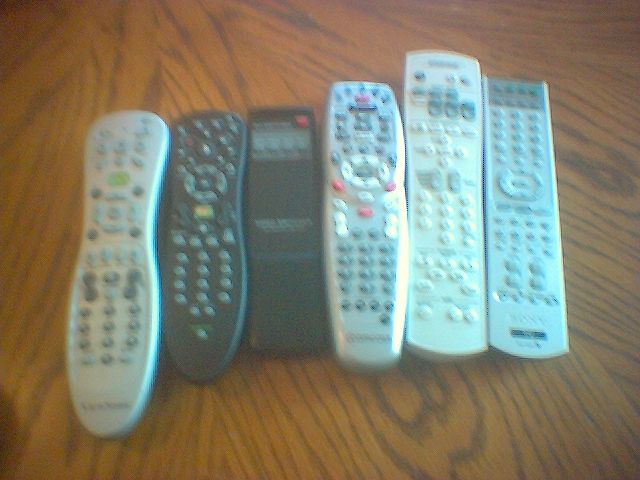The blurry, low-resolution landscape photograph depicts a collection of six remote controls of varying types, lined up side-by-side on a dark oak wooden surface with noticeable black striations running towards the back left and downwards. The remote controls are not perfectly aligned and vary in length, shape, and color. The lineup begins with a silver remote shaped somewhat like a bowling pin. Next, there is a black remote akin to those used for cable boxes. The third remote, in black, is distinctive with only about five buttons concentrated at the top, leaving the bottom mostly empty. The final three remotes are predominantly silver, with the fourth being a universal remote featuring numerous buttons. One of the remotes has an LCD display. Despite their differences, all the remotes share the characteristic of resting on the glossy wooden surface, which contributes to the overall blurred and poorly captured quality of the image.